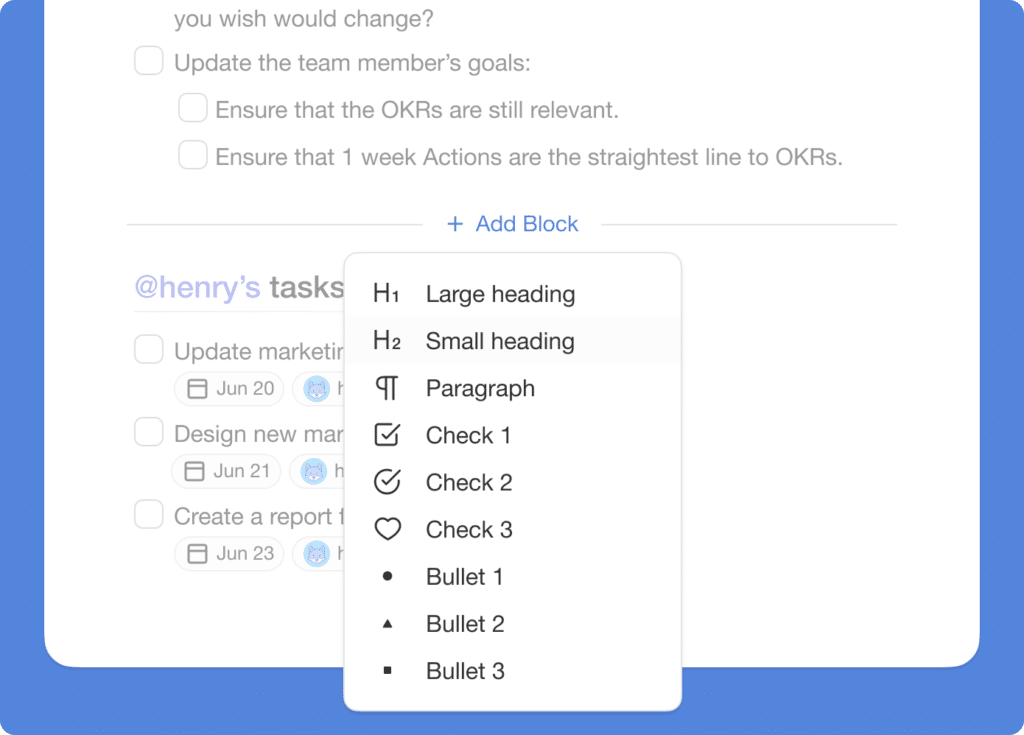This screenshot features a predominantly blue background in a rectangular format, wider than it is tall. Within this blue rectangle, there is a smaller white rectangle, although its top portion is cropped, causing some of the text to be cut off. Inside the white section, in grayish text, a message reads, "You wish it would change." Below this message, a series of actionable items are listed, including "Update the team's members' goals," "Ensure that the OKRs are still relevant," and "Ensure that one-week actions are the straightest line to OKRs." Each item has an accompanying checkbox. 

Underneath, a blue hyperlink is labeled "Add block." Further down, a section titled "Henry's tasks" lists individual tasks such as "Update marketing [cut off], June 20," "Update new [cut off], June 21," and "Create a report, June 23." Each task also features a checkbox next to it.

On the right side, a vertical menu is open displaying text formatting options in black. These options include "Large heading," "Small heading," "Paragraph," "Check one," "Check two," "Check three," "Bullet one," "Bullet two," and "Bullet three." The bullet options consist of circle, triangle, and square icons.